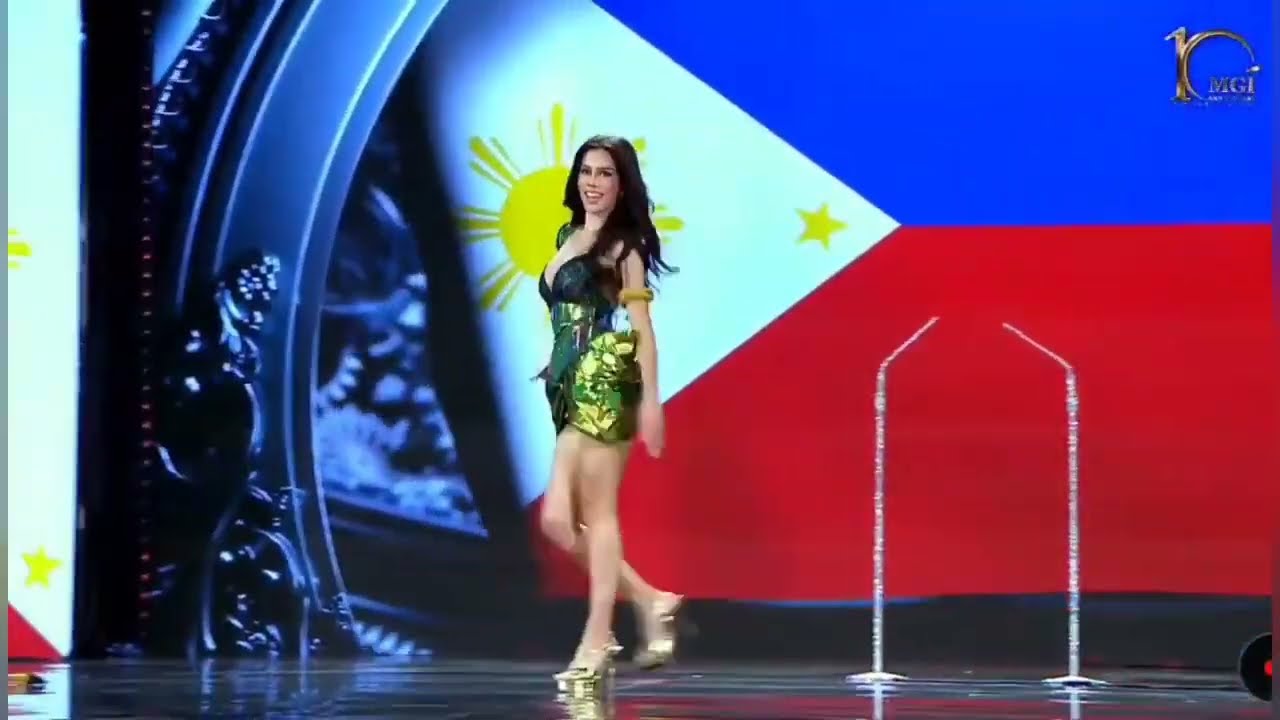The photograph depicts a young Caucasian woman, likely in her early 20s, walking across an indoor stage from right to left, with her left side facing the viewer. She gazes out at the audience with a big smile on her face. The woman wears a short, metallic dress that shimmers in shades of yellow, green, and blue, reminiscent of a beetle's iridescent shell. Her long, straight brown hair flares around her shoulders, and she is donning striking gold platform heels. Behind her, a large flag adorns the background, featuring a white triangle pointing to the right with a golden sun at its center and a smaller gold star near the triangle's apex. The upper section of the flag is blue, while the lower section is red. Additionally, there is a design pattern to the left and a logo with the initials "MGI" in the top right corner of the image.